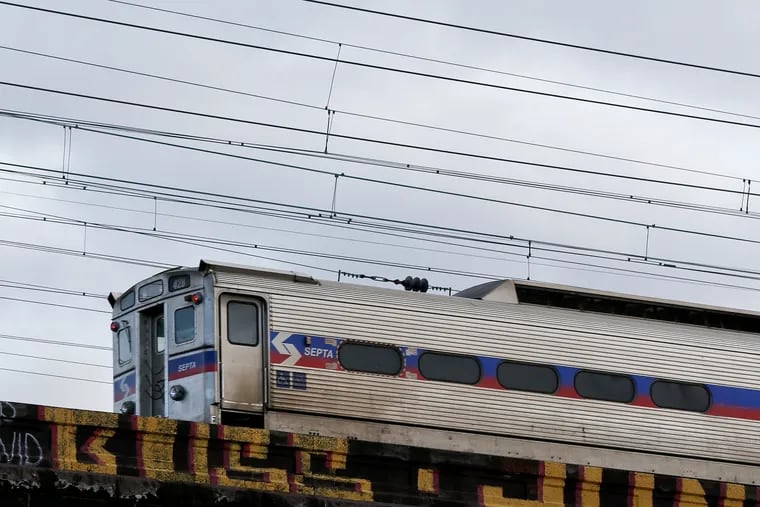This detailed photograph captures a silver and gray commuter train, possibly stationary, positioned on a track within a cityscape. The train, stretching across the bottom half of the image, features a sleek design with a red and blue stripe running horizontally along the middle, intersecting five windows. Notably, a white logo with an interlocking arrow design indicating left and right directions stands out near the front, accompanied by the text "SEPTA." The scene is set against a light blue-gray, overcast sky.

Above the train, a network of horizontal wires and cables is prominently visible, suggesting they are integral to its power system. The train's exteriors include multiple doors, including a distinct back door and side door at one end. Surrounding the track, a foundation or concrete divider is present, marked by graffiti. The graffiti, painted in large yellow letters, reads "B-U-S-S" with the letter "J" and potentially the phrase "bliss dot June." Additional smaller, white graffiti is visible to the left but remains partially obscured and difficult to decipher.